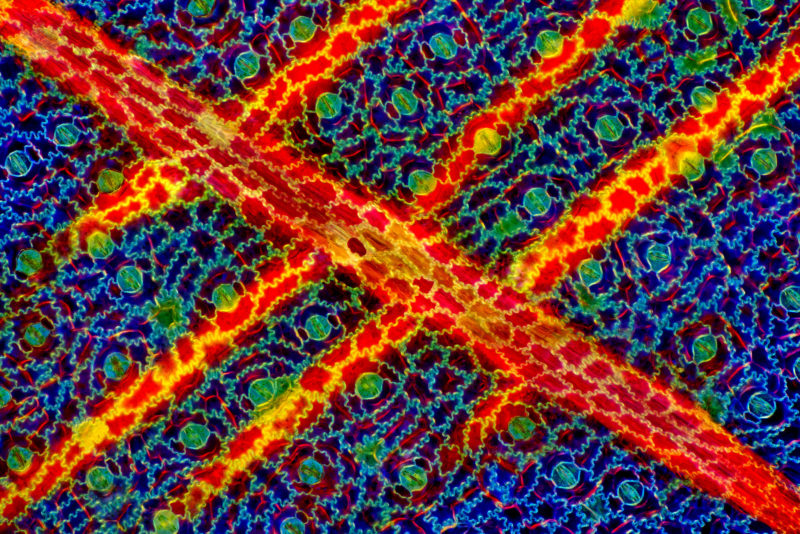This vibrant and detailed image resembles an abstract painting or colorful drawing. Dominating the composition is a dynamic pathway resembling snake-like skin that extends diagonally from the top right to the bottom left. This pathway, adorned with red, yellow, and occasional orange shapes, features multiple offshoots branching perpendicularly in the same color scheme. These vivid pathways contrast strikingly against the background, which is a rich tapestry of blues and greens. The blue areas vary in shade from light to dark, interspersed with numerous green, irregularly shaped circles and uneven dots. The overall effect is a complex, almost cellular appearance, punctuated by many squiggles and intricate designs, creating a mesmerizing fusion of organic patterns and vibrant hues.